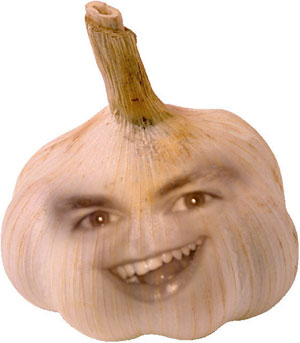The image depicts an off-white, slightly grayish bulb of garlic with its dark yellow, somewhat dirty stem still attached, set against a plain white background. The garlic appears close-up, revealing individual vertical fibers running down its skin and showing a few black spots likely from soil remnants. Imposed on the garlic is a digitally-created face, featuring a pair of dark eyebrows, two sets of eyes staring straight ahead, and an open mouth, complete with visible teeth and even a tongue. The expression on the face could be interpreted as either happy or mocking, giving the garlic a humorous, meme-like quality.